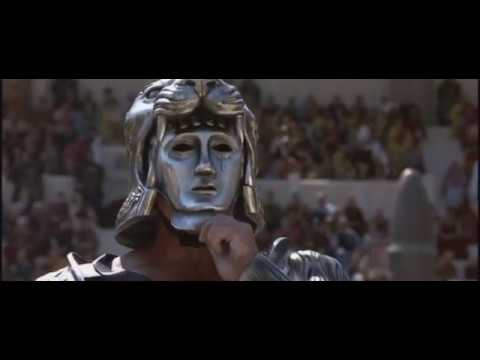This screenshot from the movie "Gladiator" features a man clad in elaborate metallic armor, notably a distinguished helmet that combines a human face mask with a lion's head on top. The man, whose neck is the only visible skin, is seen touching the chin area of his mask with his left hand, as if either adjusting or removing it. The helmet and armor, crafted from a white-gray metal, cover his shoulders and upper body. The scene takes place in an ancient arena, where two levels of stone bleachers, packed with spectators, are faintly visible behind him. The image is characterized by a thick black border at the top and bottom, with a curved arrow-shaped pillar visible at the lower right, contributing to the historic ambiance of this dramatic moment.